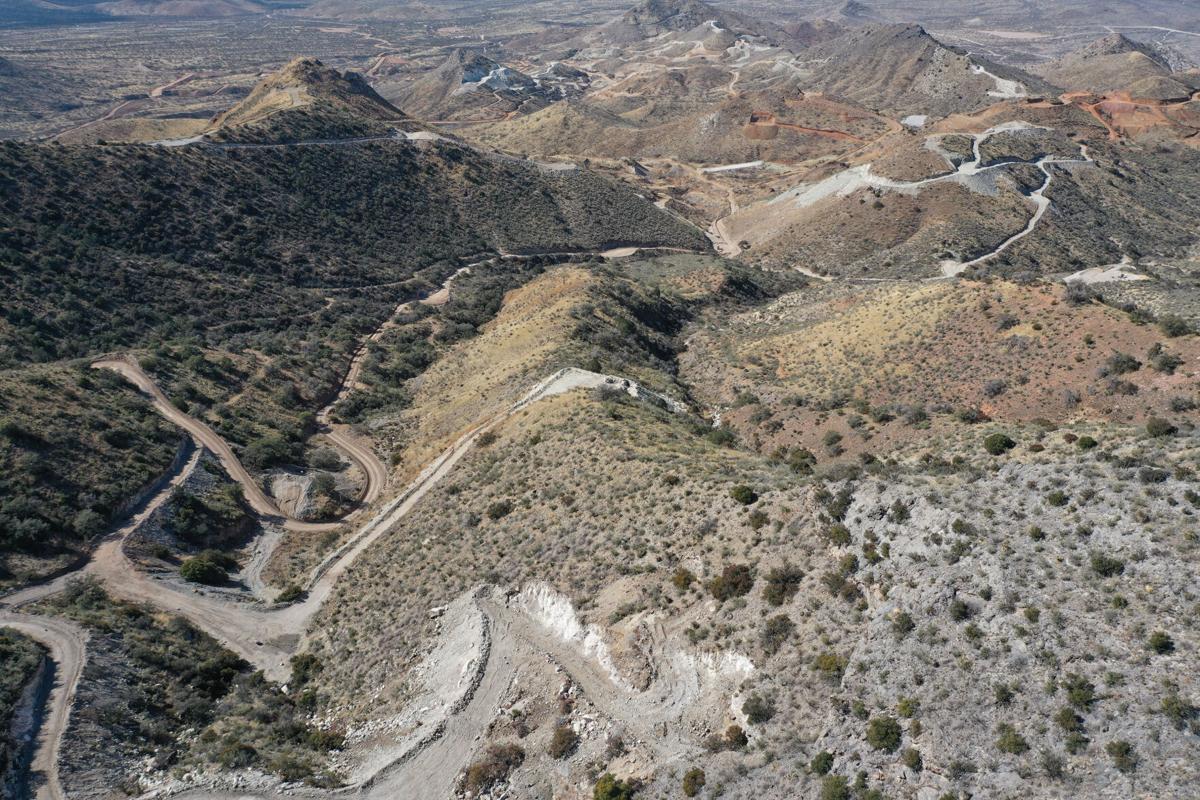This is an aerial photograph of an expansive desert and mountainscape, showcasing a desolate yet intriguing natural landscape. The primary colors in this photograph are dusty green, gray, and various shades of sand. The terrain is dominated by undulating mountains that stretch into the distant background, creating a sense of vastness. Sporadic patches of dry vegetation, such as shrubs and some green trees, are scattered haphazardly across the mountains, contrasting with the predominantly brown and arid ground. Winding dirt trails, likely meant for mountain biking or dirt biking, weave their way through the scene, emphasizing the rugged and inaccessible nature of this environment. The perspective from a high vantage point, possibly the top of one of these mountains, grants a sweeping and detailed view of this stark and barren landscape.